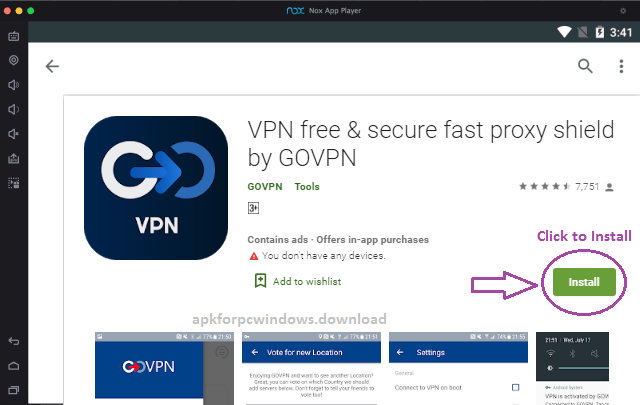The image is a screenshot of a website displayed on a digital interface. At the top, there is a header with a black background, featuring the text "Nox App Player." The word "Nox" is written in blue, while "App Player" is in white. On the far left of this header, three circular dots are visible: a red dot, a yellow dot, and a green dot.

Below the header, the status indicators for cell phone strength and Wi-Fi strength are displayed, with full Wi-Fi signal shown. An icon with a line through it (indicating a possible muted or disabled feature) and a battery meter showing a charge level are present alongside the time indicator of 3:41.

The next section on the screen has a white background, with a left-facing arrow on the right side, while a search icon and a menu icon with three dots are on the far right. Beneath this, there is a box containing the logo for a VPN application. The logo features a design with a white 'C', a blue arrow, and a blue 'C' reversed from the white 'C'.

The title within the box reads "VPN Free & Secure - Fast Proxy Shield" by GOV PN. Detailed information about the VPN service follows, and a prominent green 'Install' button with white text is enclosed within a purple circle. Above this purple circle, a purple arrow points to the 'Install' button, with the text "Click to Install" above the arrow.